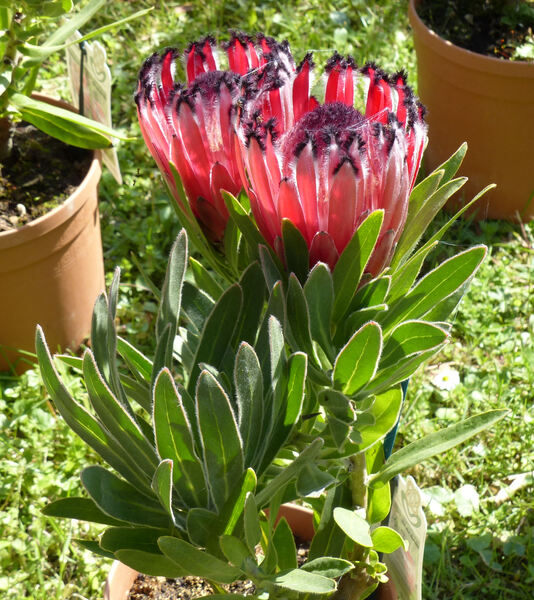This outdoor photograph captures a striking close-up of a captivating flower with green, furry, oval leaves sticking upward. The flower itself is a stunning focal point, featuring tulip-like petals that are pinkish with purple tips and fuzzy purple insides, resembling claws opening towards the sky. Surrounding this central flower are two beige terracotta pots filled with soil. The pot on the left, located toward the middle of the image, has identifiable green leaves emerging from it, while the pot on the right in the top corner shows only the soil. Both pots seem to be placed on a grassy lawn, hinting at a sunny day. A sign attached to one of the pots adds a touch of intrigue, as it's facing away from the camera and remains unreadable. The photograph's well-crafted composition and vivid details highlight the unique beauty of the plants within this garden-like setting.